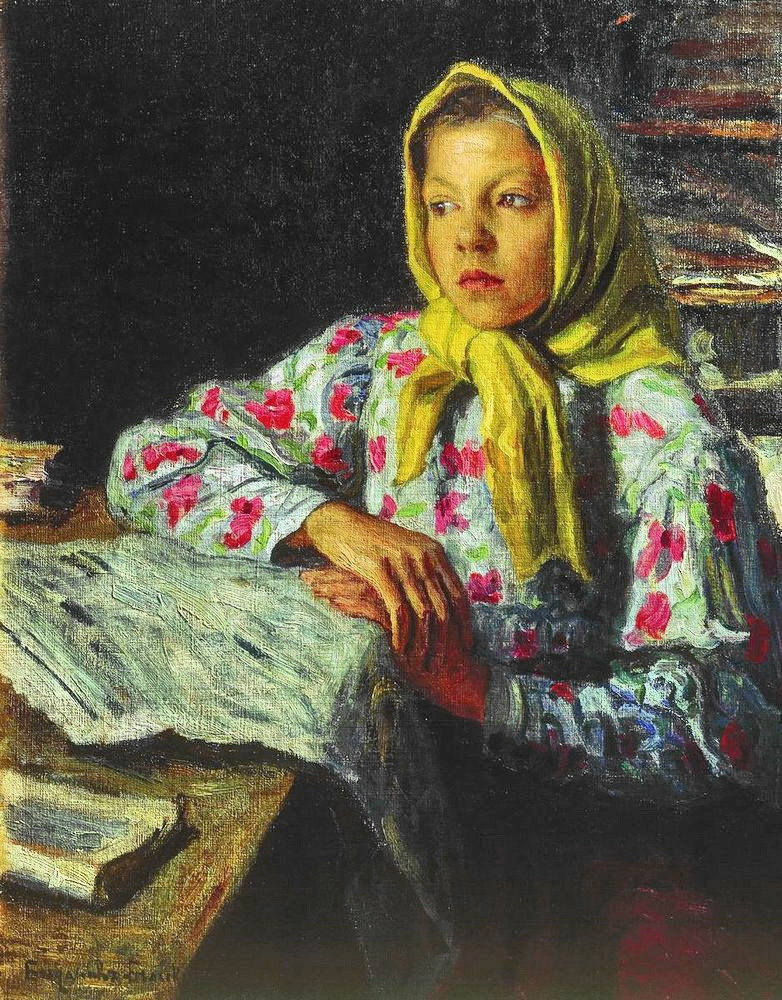The image depicts a young Caucasian woman with light-colored hair and red lips, seated at a wooden table. She is dressed in a white long-sleeved shirt adorned with pink flowers and green leaves. A yellow scarf is wrapped around her head completely. The woman has a pensive and contemplative expression, her brown eyes gazing off to the side. Her right forearm rests on the table, with her right hand placed gently over her left hand, which grips the edge of the wooden surface. In front of her, on the table, lies a piece of paper or book with indistinct markings, hinting at recent reading or writing. The background is dark, emphasizing her thoughtful demeanor.